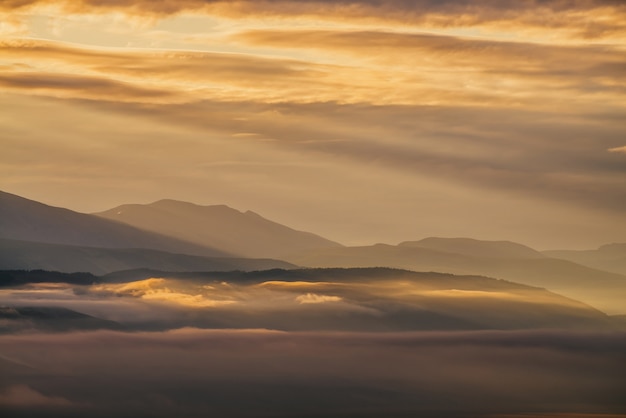This photograph captures a serene mountainscape bathed in the soft, warm light of a setting sun. The sky is a tranquil blend of oranges, peaches, and grays, with wispy clouds illuminated from behind. The upper clouds form delicate streaks of color, while lower foggy layers roll across the scene, creating an ethereal atmosphere. In the background, the mountains stand in shadow, their silhouettes painted in deep purples and grays, blending smoothly into the mist and sky. The entire landscape is suffused with an almost otherworldly glow, its hues reflecting the sunset in a harmonious gradient. This beautiful, tranquil scene, with its interplay of light and shadow, evokes a sense of peace and could easily be a perfect wallpaper or desktop background.